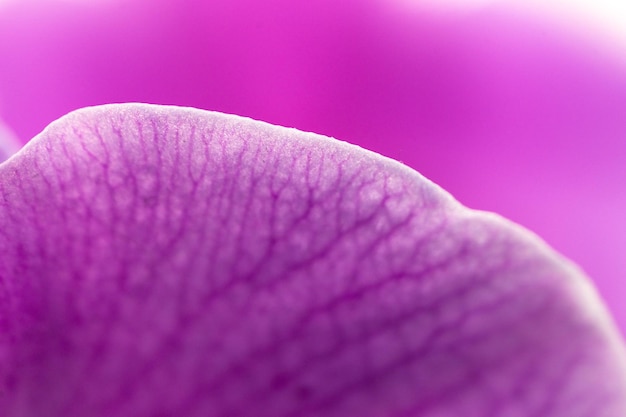This image is an intensely zoomed-in, possibly microscopic photo of what appears to be a plant leaf or petal, showcasing a variety of artificial colors. The focal point is a semi-translucent structure with distinct dark purple veins intricately spread throughout, creating a striking visual contrast. The object is bathed in a highlighted light pink rim that enhances its delicate, ethereal quality. The blurred background is a wash of purples, pinks, and whites, contributing to a surreal, almost dream-like atmosphere. The image's color palette, including magenta and white halos, adds to its artistic and otherworldly appearance, making it difficult to definitively identify the subject.